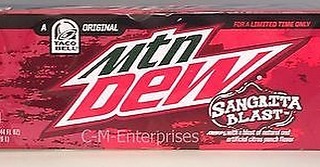This photograph showcases a case of Mountain Dew's limited edition Sangrita Blast. The packaging prominently features a vibrant red design, drawing immediate attention to its unique flavor. The label on the case abbreviates Mountain Dew as "MTN DEW," aligning with the brand's trend of modern shorthand. Additionally, the top left corner of the case bears the Taco Bell logo, signifying that this particular flavor is a Taco Bell Original. To the left of the Taco Bell symbol is the letter "A," and to its right, the word "Original," reinforcing the exclusive collaboration between Mountain Dew and Taco Bell to create the Sangrita Blast flavor. The detail captured in this photograph not only highlights the distinctive nature of the Sangrita Blast but also emphasizes its culinary connection to Taco Bell.